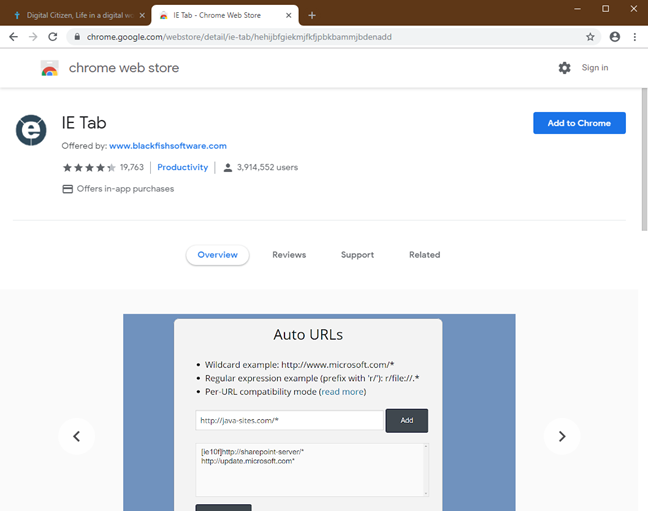The screenshot captures the Chrome web browser displaying two tabs. The inactive tab is partially titled "Digital Citizen, Life in a Digital...," with the rest of the title cut off. The active tab showcases the "IE Tab" extension on the Chrome Web Store. The primary content of the screenshot focuses on the IE Tab homepage, an extension provided by blackfishsoftware.com. 

Prominently displayed, the extension boasts 19,763 ratings, is categorized under productivity apps, and has over 3.9 million users. At the bottom center of the screen, navigational tabs titled "Overview," "Reviews," "Support," and "Related" offer further insights into the extension. Below these tabs, a series of images provide additional information regarding the extension’s features and functionality.

In the top right corner, a noticeable large blue button with white text reads "Add to Chrome," inviting users to install the extension for enhanced browsing capabilities.